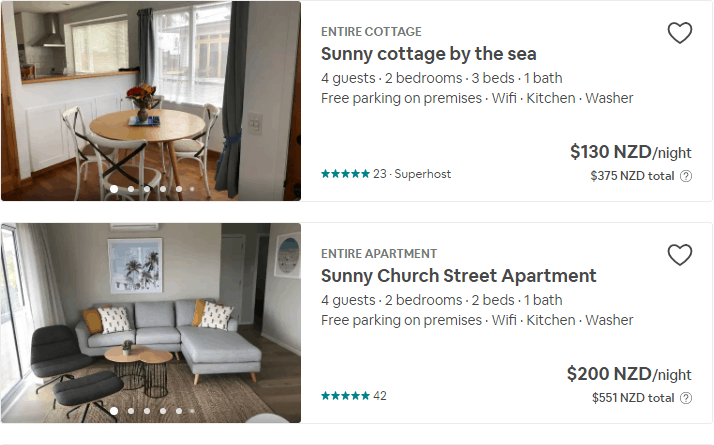The image showcases two separate accommodations: a cottage and an apartment, each complete with details about their interiors and amenities. 

**Top Section:**
- **Accommodation:** Sunny Cottage by the Sea
- **Description:** The image includes a cozy interior photo on the left, complemented by a detailed description on the right.
- **Details:**
  - **Capacity:** 4 guests
  - **Rooms:** 2 bedrooms, 3 beds
  - **Amenities:** 1 bathroom, free parking on premises, Wi-Fi, kitchen, washer
  - **Pricing:** 130 NZD per night

**Bottom Section:**
- **Accommodation:** Sunny Church Street Apartment
- **Description:** An inviting photo of the apartment's interior is displayed on the left, with relevant details listed on the right.
- **Details:**
  - **Capacity:** 4 guests
  - **Rooms:** 2 bedrooms, 2 beds
  - **Amenities:** 1 bathroom, free parking on premises, Wi-Fi, kitchen, washer
  - **Pricing:** 200 NZD per night

The information provides a comprehensive overview, helping potential guests choose the accommodation that best suits their needs.